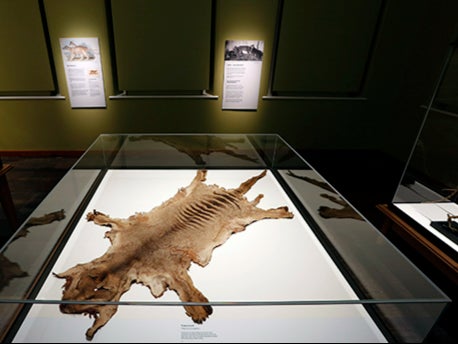This photograph captures a dimly lit museum exhibit showcasing an animal hide inside a top-down glass display case. The hide, possibly from a mammal, is laid out flat, revealing its unique features: a brown head, a lighter brown body with a dark brown stripe running down the back, four legs, and a long tail. The texture of the hide appears mostly smooth, with some roughness along the back vertebrae. The bright white base of the case illuminates the hide, drawing attention to its intricate details. Surrounding the case, the background remains dark, but we can see the corner of an adjacent glass display and two backlit informational signs. One sign features an animal image with accompanying text, while the other contains a black-and-white image and additional writing. A set of railings can also be observed in the background, contributing to the exhibit's overall setting.